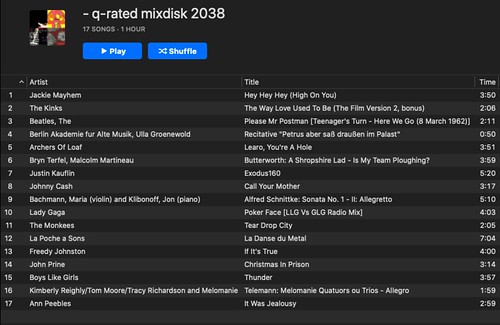Digital collage featuring various music artists and their song titles:
1. **Jackie Mayhem** - "Hey Hey Hey (High on You)"
2. **The Kinks** - "The Way Love Used To Be (Film Version Bonus Track)"
3. **The Beatles** - "Please Mr. Postman"
4. **Berlin Academy** - "For Her Alti Music Recitative"
5. **Archers of Loaf** - "Zero, You're a Whole Number"
6. **Bryn Terfel** - "Butterworth"
7. **Justin Kauflin** - "Exodus 160"
8. **Johnny Cash** - "Call Your Mother"
9. **Maria Backman** (featuring Alfred Shantiki) - "Sonata No. 1"
10. **Lady Gaga** - "Poker Face"